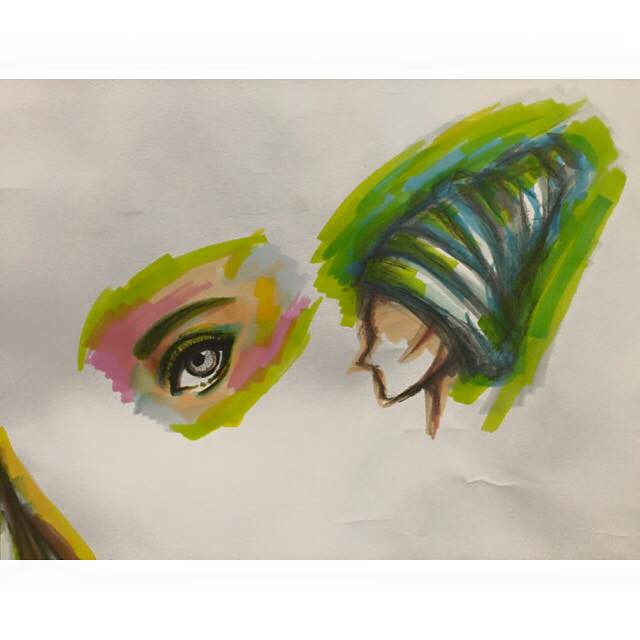This abstract artistic image, rendered in marker, showcases a vibrant use of colors ranging from white, pink, tan, and green. The artwork appears on slightly wrinkled white paper, adding a textured dimension to the piece. In the bottom left corner, brown and yellow lines make an appearance, though they are partially cut off, leaving their full form to the imagination.

Central to the composition is a distinctly rendered eye. Its white sclera takes on a grayish tone, while the pupil stands out vividly. The eye is framed by detailed eyelashes and highlighted with green eyeshadow. A matching green eyebrow arches above, completing the expressive eye.

Surrounding the eye is a medley of skin-tone hues, incorporating tan and pink, interspersed with areas of lime green. Adjacent to this is what appears to be the side profile of a face, from which emerges a swirling, cone-like structure. This striking element spirals in mixed shades of white, green, and blue, featuring additional green and light blue striping that adds to the dynamic movement of the image.